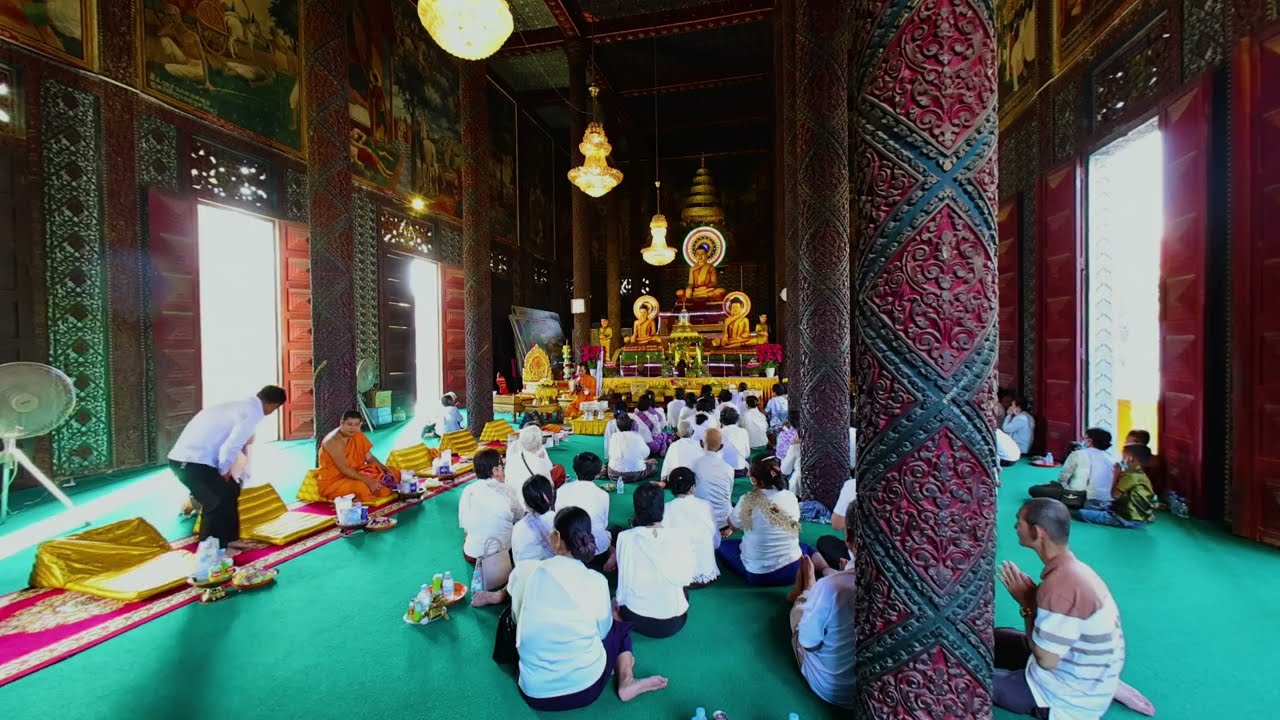The image depicts the inside of a vibrant and ornate prayer hall, richly decorated and filled with devotees. At the far end of the room, elevated on a platform, sit three large golden Buddha statues. The center statue is the largest, with two slightly smaller ones on either side. Each Buddha has a circular halo behind their head and is seated cross-legged, wearing yellowish robes.

The room is alive with color. The walls are red and teal, adorned with intricate, scroll-like designs, and the pillars exhibit beautiful blue and red decorations. The ceiling is adorned with colorful paintings. Bright light streams through open doors on both the left and right sides, illuminating the scene.

The floor, a striking teal green, is where the congregation sits, mostly wearing white shirts. The attendees are either kneeling or sitting cross-legged, many with hands clasped in prayer. Notably, on the left side, a man in white appears to be conversing with a Buddhist priest dressed in orange, who sits with his arms wrapped around his left knee.

To the far left, a red carpet runs along, leading to cushioned seating areas wrapped in gold material, possibly designated for more important individuals. This area also features trays of food in front of the mats, indicating a special arrangement. Additionally, a pedestal fan is visible on the left.

The overall atmosphere exudes a sense of reverence and cultural richness, capturing the essence of a devotional gathering within an elaborately adorned Buddhist temple.